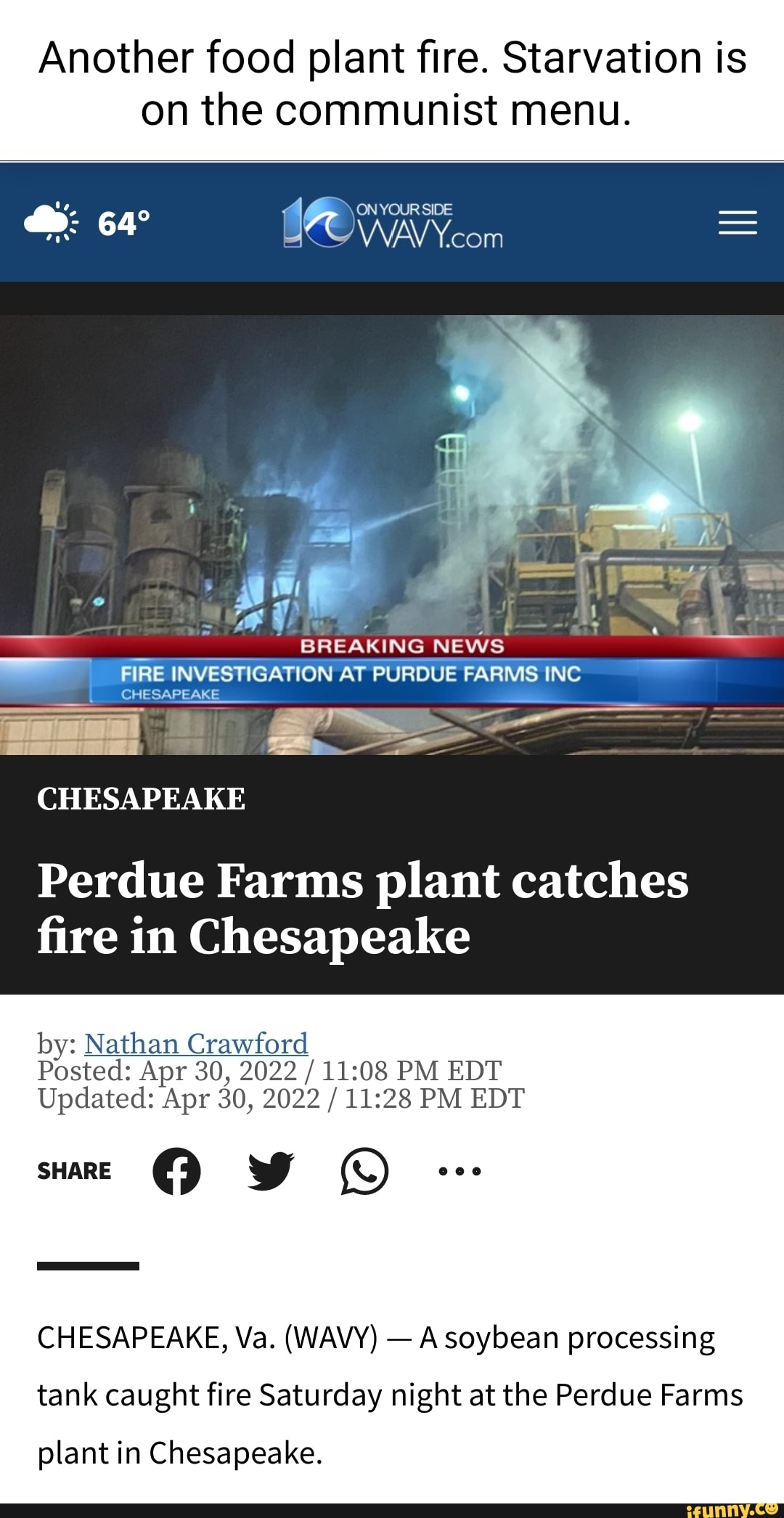Title: "Breaking News: Fire Erupts at Purdue Plant in Chesapeake"

Caption: In this dramatic image, a screenshot captures the chaos of a news report about a significant event. The image features a bold headline with black text on a white background, stating: "I have food, planet, fire, starvation, on the communist menu." Below this headline is a fragmented news article discussing a fire at a Purdue plant in Chesapeake. The central portion of the image shows a news broadcast screenshot with the breaking news alert, "Fire and desolation approved," followed by visuals of a blazing plant at night with smoke illuminated by various lights. The top left corner indicates the weather at 64 degrees, while the middle section of the screen reads "sitting curbside" alongside the logo "wavy.com" and three horizontal lines representing settings. The article is authored by Nathan Crawford and notes the incident was posted on April 30th, 2022, at 11:08 PM EDT and updated at 11:28 PM EDT. Social media icons for sharing on Facebook, Twitter, and a phone icon appear as well, just above the beginning sentences of the article which starts with "Chesapeake, Virginia."